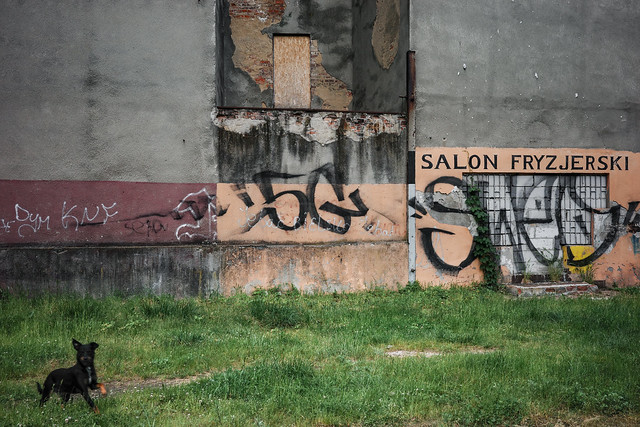In the image, a black dog with perked ears is positioned on the lower left side, gazing directly at the camera. The foreground features a patch of uneven, wild grass. The main focus is a large, weathered concrete wall marked with various forms of graffiti. On the far left, a crimson section with white spray paint is visible, and below that, the blackened, aged stone is apparent. The central area of the wall appears damaged, with what looks like a discolored, rusted door covered by plywood. Above this deteriorated section, the graffiti "5G" is spray painted, with a dull yellow background beneath it. Moving towards the right, black font reading "Salon Fresjerski" is prominently displayed on a light orange background. The wall further shows signs of wear and multiple layers of graffiti, suggesting a long history of tagging. Overall, the combination of the unkempt grass, the varied graffiti, and the deteriorating wall paint a picture of a neglected urban area.